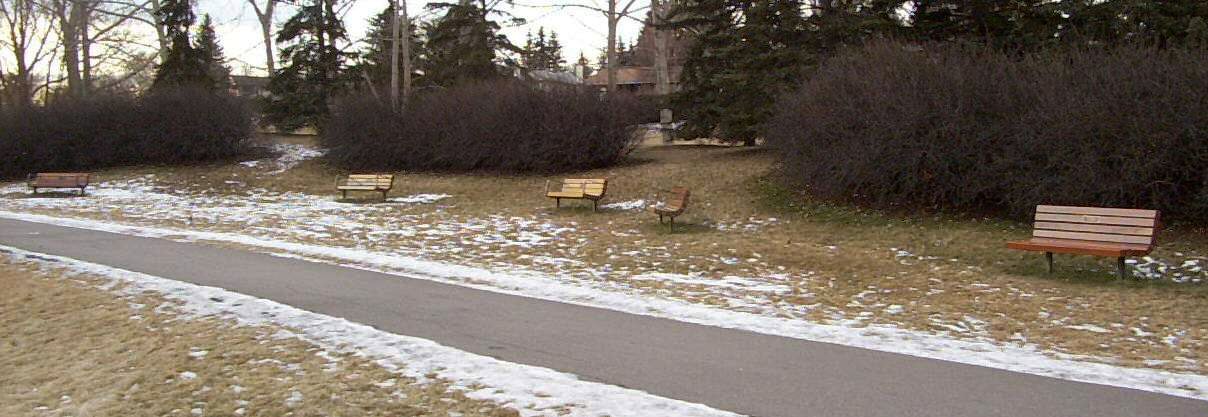This wide-angle photograph of a park walkway, taken during the daytime in winter, captures a serene scene characterized by a central asphalt path flanked by grassy areas interspersed with patches of melting snow. The park is quiet, with the grass appearing dormant, indicative of the season. The walkway is lined with wooden benches on the right, positioned every few feet; these benches vary in shades of brown, with some lighter and others darker. Additionally, a unique reclining chair stands out among them. To the right, dense, tall, dark trees with wide branches create a thick backdrop, and in front of these are tall pine trees and some dark bushes. At the far end of the park, a stone tower or brown building is barely visible, adding a distant focal point to the tranquil setting.